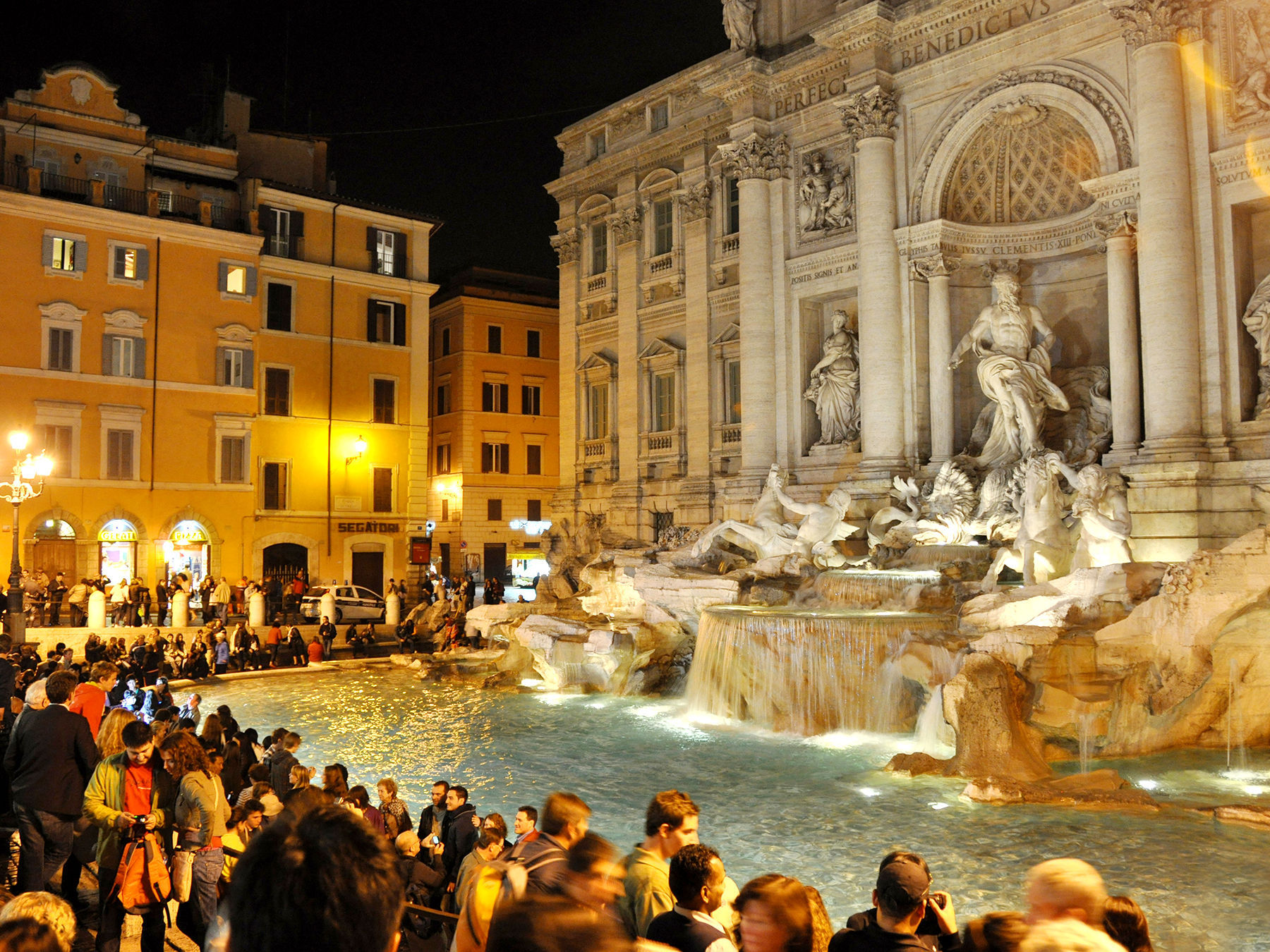The photograph captures a vibrant, bustling public area at nighttime dominated by an ornate, historical building with a large, elaborate fountain that features a waterfall design flowing into a sizeable pool at the foreground. The impressive edifice, reminiscent of a white castle or cathedral, boasts intricate Greek-style statues on its façade, including detailed reliefs of figures appearing to be in a state of merrymaking. This scenic spot is aglow with excellent illumination, enhancing the building’s decorative elements and antique-style streetlights that add to the atmosphere. Text etched on the building reads "Perfect Benedictus," providing a hint of its possible cultural or historical significance. The scene is teeming with life, with a large crowd gathered around the fountain and pool, capturing photos, socializing, and enjoying the lively ambiance of what seems to be a major center of commerce. Amidst the milling crowd and a car parked on the street, the image offers a picturesque and dynamic snapshot of nighttime urban life.